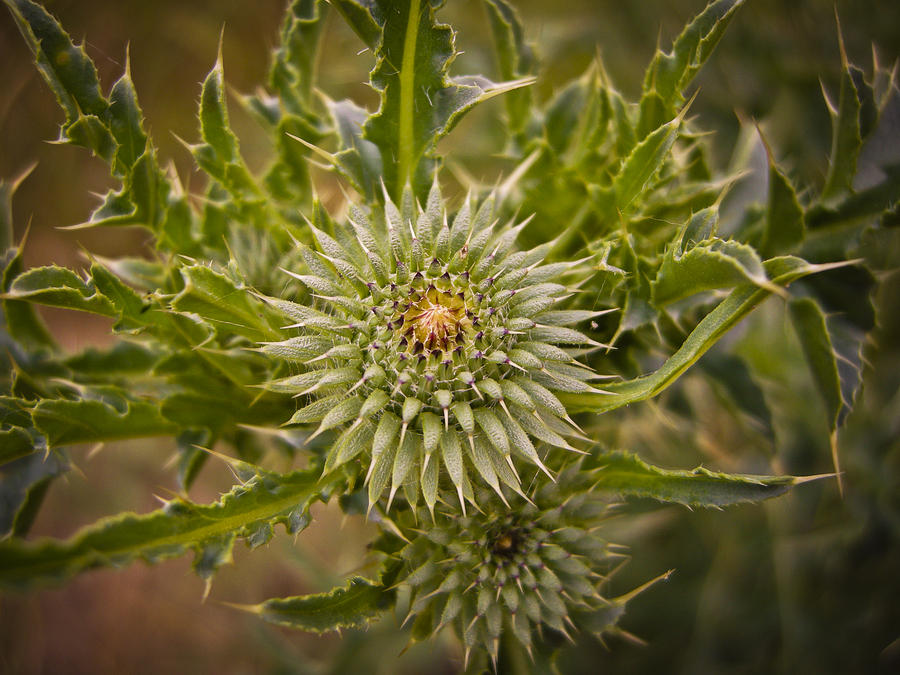This extremely close-up photograph captures a strikingly spiky desert plant with distinct, sharp leaves that are predominantly green adorned with light green veining and tipped with intimidating maroon-hued prickers. The plant features two prominent, ball-shaped central structures that are also spiky, with the upper ball displaying a yellow center fading into a light brown as the spikes, increasingly smaller, converge towards the middle, giving an impression of an unfurling bloom. The lower spiky ball has a less vibrant tan center. The blurred background consists of earth tones—browns and dark hues—implying a dry, dusty environment that softly recedes into the distance and enhances the surreal, almost alien, appearance of the plant.